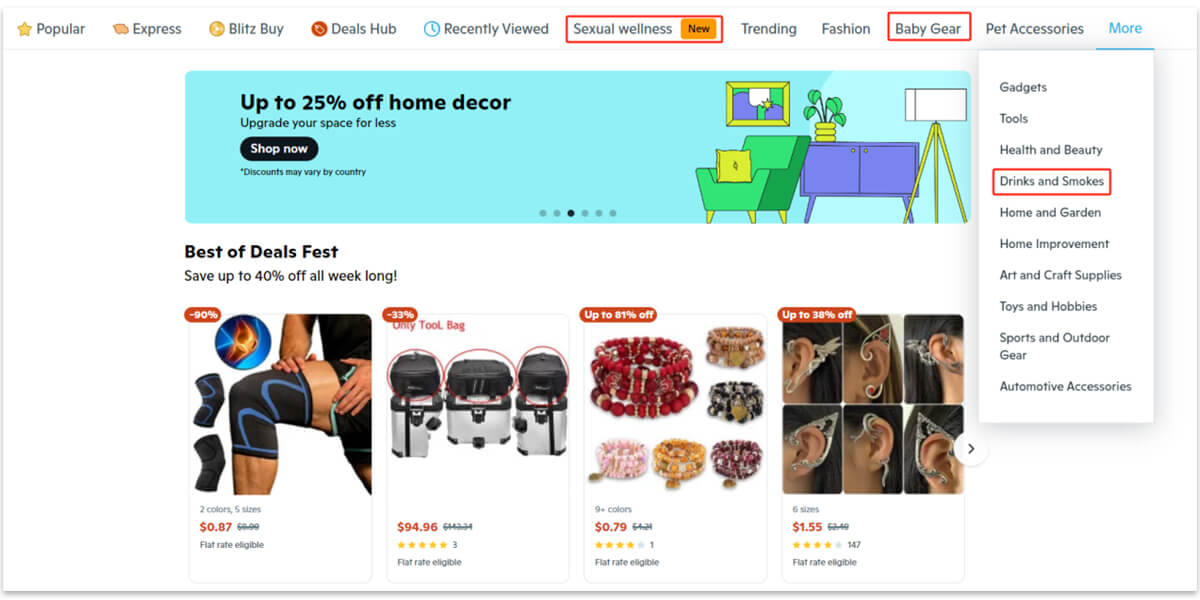The image depicts a comprehensive e-commerce website featuring a diverse array of products. At the top, there's a prominent search bar accompanied by tabs for "Popular," "Express," "BlitzBuy," "Deals Hub," and "Recently Viewed." Additionally, there is a "Sexual Wellness" category highlighted with a red box, further accentuated by an orange 'New' label. Other categories include "Trending," "Fashion," and "Baby Gear" (also within a red box), followed by "Pet Accessories."

Upon expanding the "More" hyperlink, further categories such as "Gadgets," "Tools," "Health and Beauty," and "Drinks and Smokes" (highlighted with a red box) become visible. Additional sections include "Home and Garden," "Home Improvement," "Art and Craft Supplies," "Toys and Hobbies," "Sports and Outdoor Gear," and "Automotive Accessories."

A banner at the top promotes a special sale with up to 25% off on home décor items, encouraging shoppers to upgrade their spaces at reduced prices. The banner notes that discounts vary by country and includes a "Shop Now" button.

Prominent deals displayed on the site include a knee support priced at $0.87, a cooler bag for $94.96, bracelets at $0.79, earrings designed for the upper ear priced at $1.55, and another set of earrings for traditional piercings at $1.55.